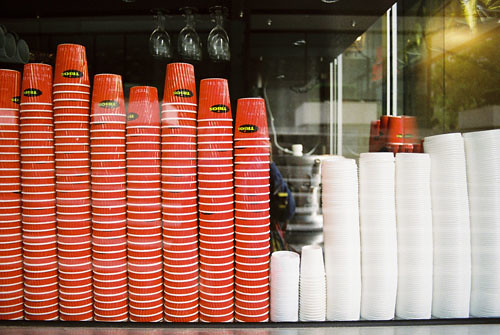In the image, we see the interior of what appears to be a cafe or coffee shop, viewed from outside through a window. Dominating the scene are eight towering stacks of red cups, each adorned with an unreadable word in yellow lettering inside a black oval. To the right of these are five stacks of to-go lids, alongside two stacks of smaller cups with matching lids. Further in the background, we observe machinery likely used for preparing drinks, and overhead, wine glasses are suspended from the ceiling. On the right side of the image, there's another window, contributing to the sense of transparency and openness of the space. The careful organization and visibility of the cups and lids raise a question about their sanitary condition.